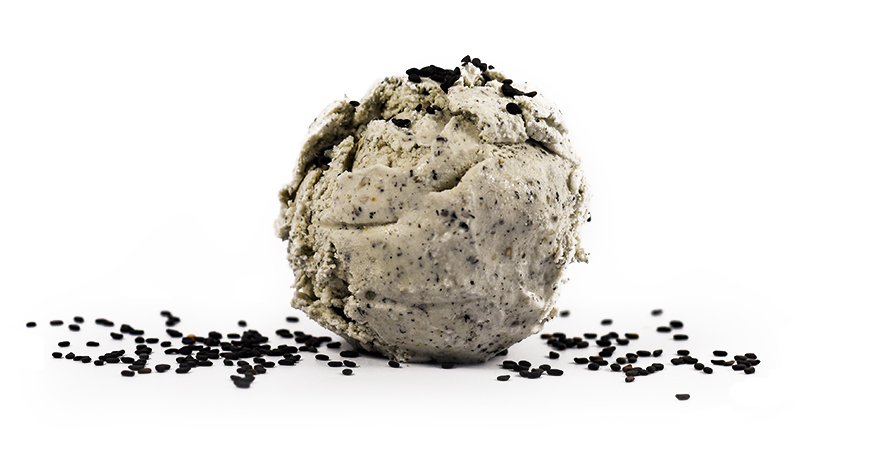The image is a color photograph showcasing a detailed, round scoop of chocolate chip ice cream set against a white background. The ice cream is creamy white with notable black speckles of chocolate chips throughout, giving it a textured and grainy appearance. The scoop has irregularities with melting layers on the sides, including a few ridges and indentations that add to its realistic depiction. A dusting of chocolate sprinkles, also referred to as jimmies, is scattered on top and around the scoop, with a heavier concentration on the left side. These sprinkles extend horizontally on either side of the ice cream, contributing to the overall presentation. Overall, the photograph exemplifies realistic food photography with its intricate details and textural intricacies.